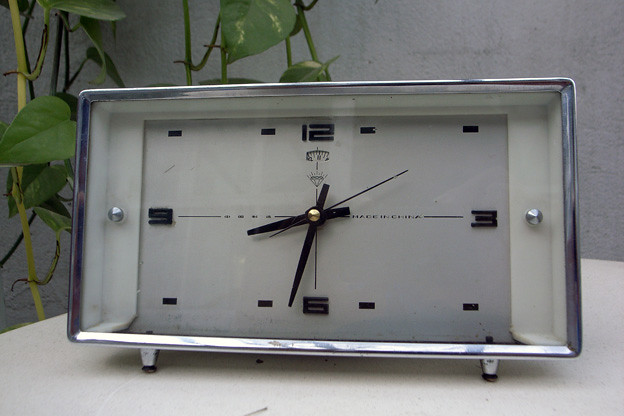The image features a retro-style, rectangular alarm clock with a silver metallic frame and a slim profile. The clock stands on two short metal legs, each fitted with black circular feet. The white clock face is protected by a glass cover and is slightly recessed into the frame. Large black numbers mark 12, 3, 6, and 9, while the remaining positions are indicated by black dash marks. The area around 12 is decorated with additional small dashes. The hour and minute hands, both black, are secured with a gold screw, and a separate second hand is also visible. The clock sits on a white or off-white wooden surface, in front of a gray stone wall with visible imperfections, adding to the textured backdrop. Green vines with leaves are creeping along the stone wall behind the clock, enhancing the rustic aesthetic. There is also some indistinct writing on the clock face, including a "Made in China" label.